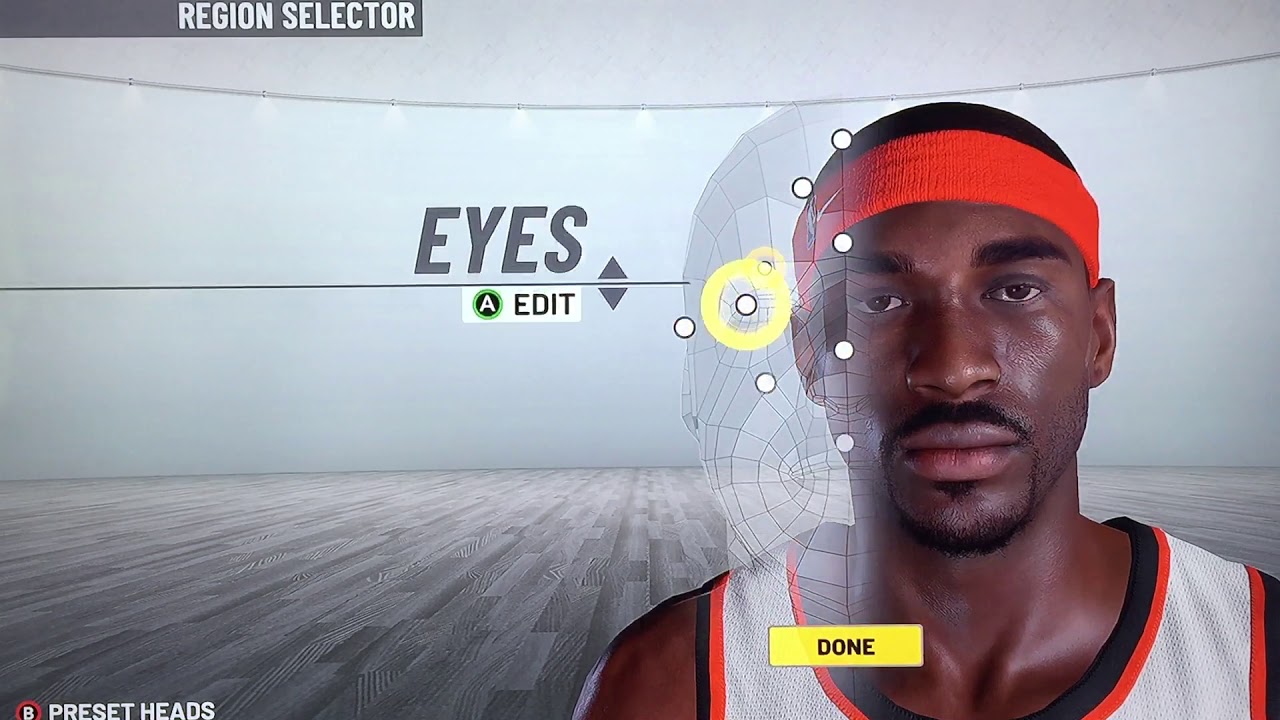The image portrays a digital rendering of a black basketball player. He is depicted wearing a red sweatband on his forehead and a white basketball jersey adorned with black and orange stripes around the neckline and arm openings. The player's face is partially overlaid with a detailed 3D mapping, showcasing a gradation effect on one side. To the left of his face, nine points are highlighted with white dots encircled in black, accompanied by two yellow circles.

Adjacent to this graphic, a rectangular bar at the bottom bears the label “Done” in black text. Above this bar, the word "Eyes" appears in large, bold letters, linked by a line to the left-hand section of the image. Flanking this line are up and down arrows. Below it, a white rectangle with a green circle is inscribed with the letter "A" and the word "Edit." 

In the upper left corner of the image, there is a gray rectangle labeled “Region Selector.” This intricate visual effectively combines elements of 3D facial mapping with interactive graphical annotations and user interface elements, likely indicating a software tool for image editing or facial recognition analysis.